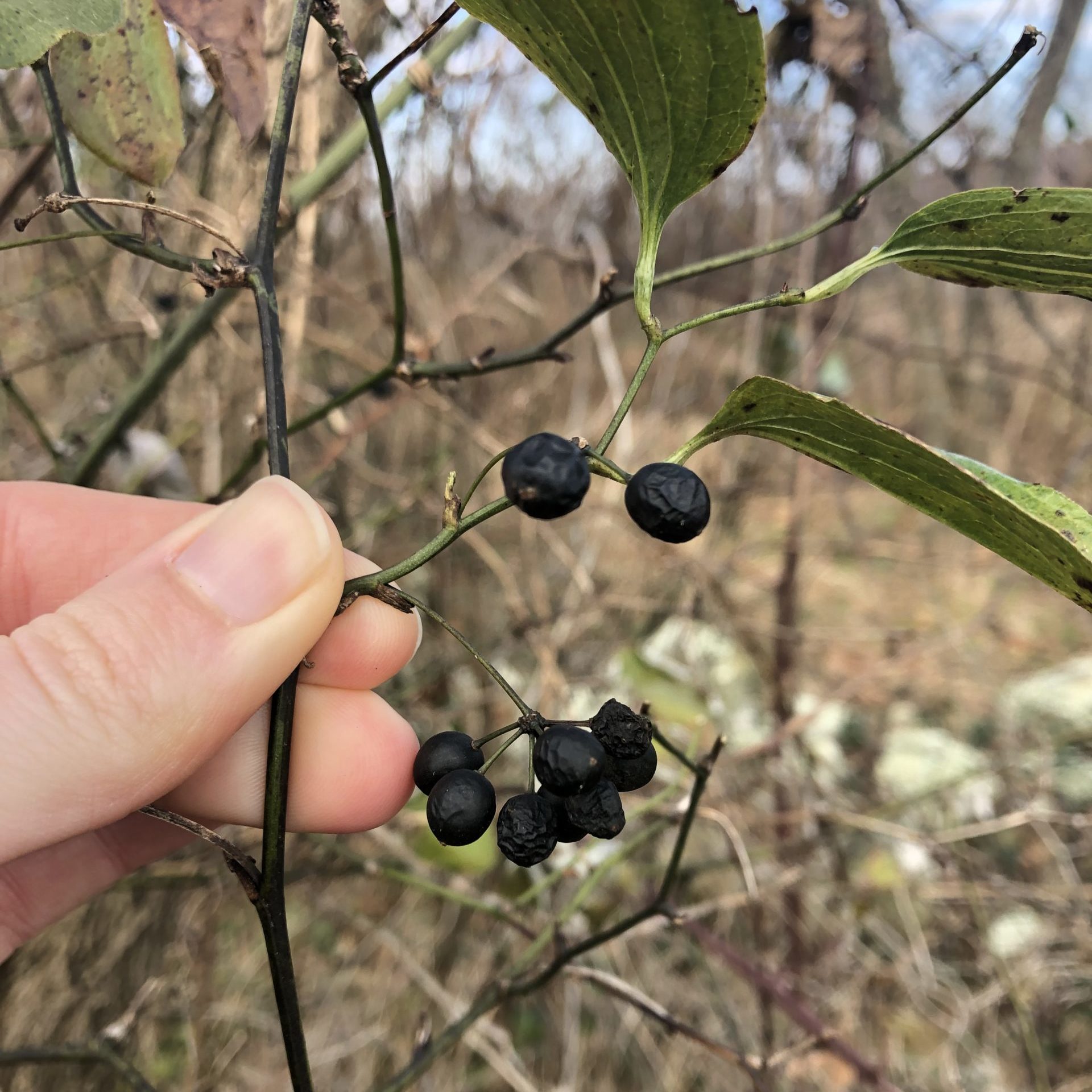The photograph captures an outdoor scene during daytime, featuring a vertically rectangular, full-color close-up of a Caucasian hand from the right side. The fingers—thumb, pointer, and middle—are holding a slender, black stem with small, shriveled black berries and a few green leaves. The background is a blurred mix of brownish tall grass, bare vegetation, and brush, with some blue sky visible at the top, enhancing the brightness and clarity of the image. The detailed focus on the hand and the stem creates a clear and crisp foreground contrast with the natural, muted tones of the out-of-focus background.